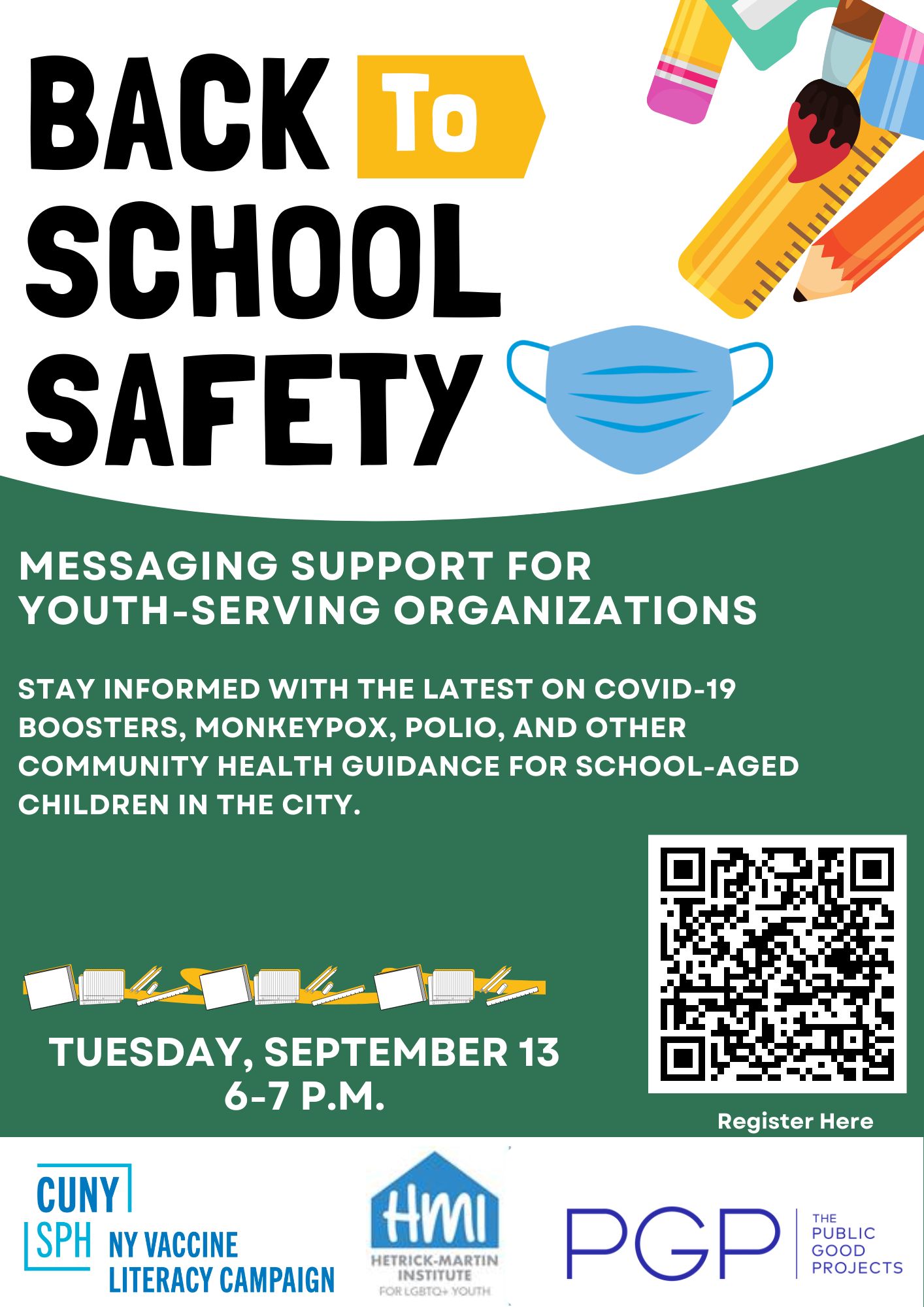This color illustration features a detailed public safety message regarding back-to-school safety. The graphic, set on a white background, has a variety of school items cascading from the top right corner. These include a yellow pencil with a pink eraser, a green sharpener, an orange paintbrush with red detailing, a blue facial mask, a gold ruler, and an orange pencil. 

In the upper left corner, black text reads, "Back to School Safety," with the word "to" highlighted in white on a gold arrow pointing to the right. Below, a green, curved panel contains a white text message: "Messaging Support for Youth-Serving Organizations." Further down, the text emphasizes staying informed about the latest on COVID-19, Monkeypox, Polio, and other community health guidance for school-aged children.

At the bottom, in the left half, the poster details the date and time for an event: "Tuesday, September 13, 6 to 7 PM." Adjacent to this, on the bottom right, is a black and white QR code labeled "Register Here." The poster also includes logos at the bottom, associated with organizations such as CUNY SPH, the New York Vaccine Literacy Campaign, HMI, and PGP.